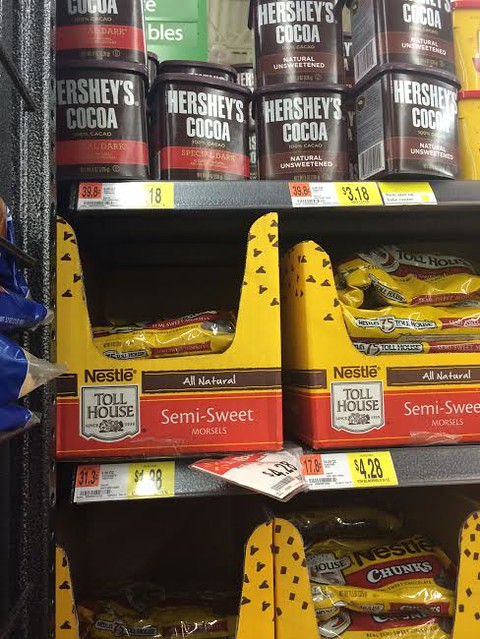A detailed image caption for the described picture:

The image is of a neatly organized section of a shelf in the baking aisle of a store, specifically dedicated to baking chocolates. The display consists of three shelves, each showcasing different types of baking ingredients. 

On the top shelf, there are rectangular dark brown containers of Hershey's baking cocoa arranged side by side. The left side of this shelf features Hershey's "Special Dark" cocoa, and the right side showcases the "Natural Unsweetened" variety.

The middle shelf is dedicated to Nestlé Toll House products, prominently displaying bags of semi-sweet morsels, which are perfect for chocolate chip cookies and other baked goods.

On the bottom shelf, there are Nestlé chunks in two cardboard boxes, indicating a more limited stock of these larger chocolate pieces. The shelf space also features a few blue bags, but these bags are only partially visible due to the angle of the photo, making it unclear what product they contain.

This organized display provides a clear and varied selection of baking chocolates, making it easy for customers to find their preferred ingredients for their baking needs.